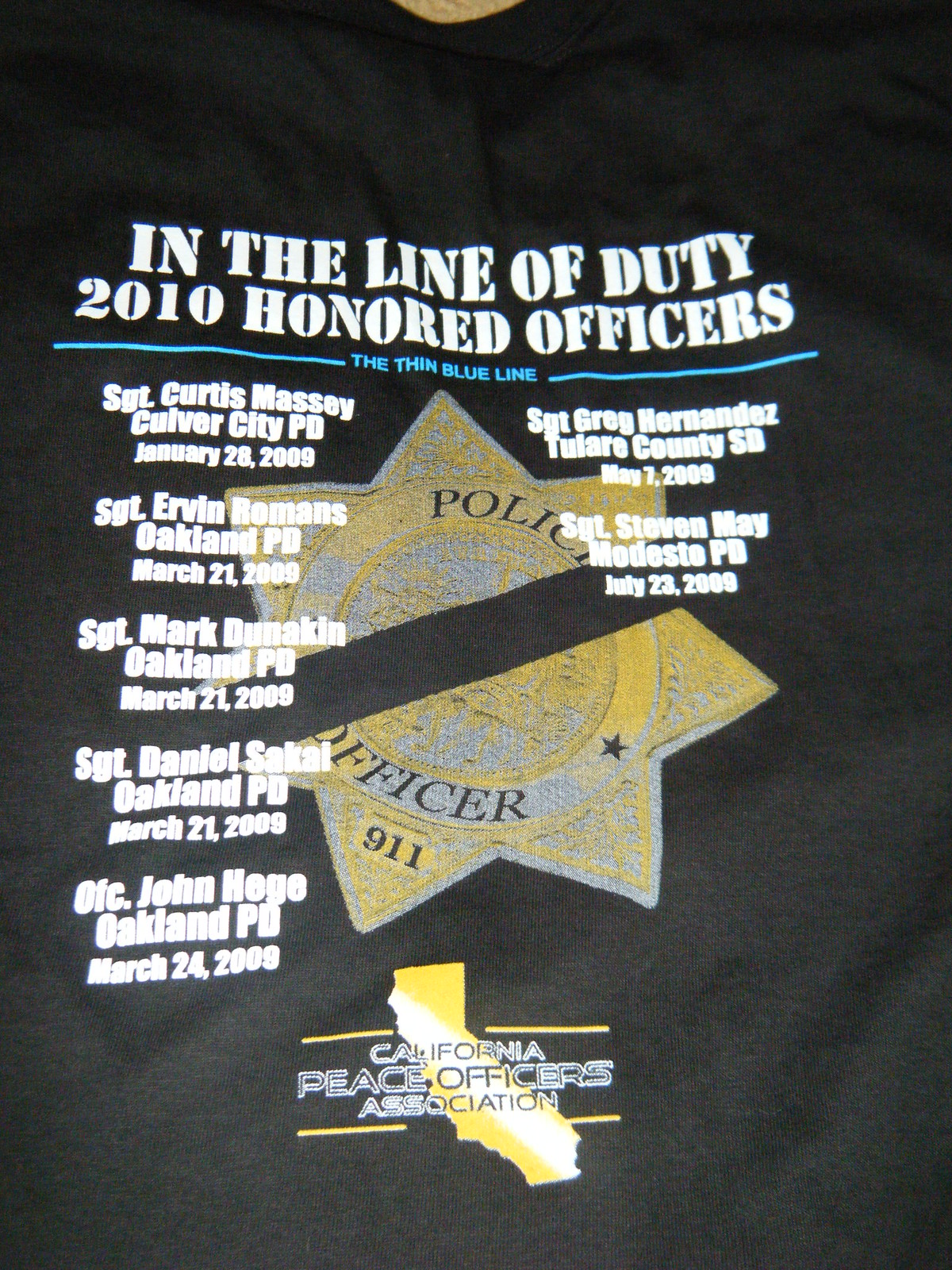The image depicts a black t-shirt laid flat, featuring a memorial design for fallen officers. The text is predominantly white, with some gold and blue accents. Dominating the shirt is a somber tribute to officers who lost their lives in the line of duty. The top section reads "In the Line of Duty: 2010 Honored Officers" in prominent block letters, flanked by thin blue lines. Underneath, the names, ranks, and departments of seven officers are listed: Sergeant Curtis Massey, Sergeant Irvin Roman, Sergeant Mark Dunnigan, Sergeant Daniel Sakal, Officer John Hedge, Sergeant Greg Hernandez, and Sergeant Stephen May, all of whom died on duty in March 2009. Centrally located is a gold and grey police shield bearing the inscription "Police Officer 9-1-1," with a black stripe running diagonally across it, symbolizing mourning. The bottom section features the logo of the California Peace Officers Association, depicting the state of California in gold with the association's name in white and black text overlaid.